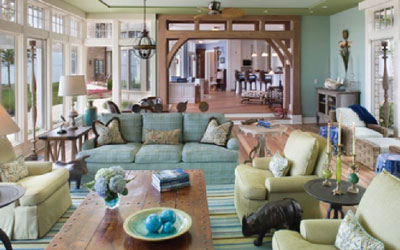The indoor daytime photograph showcases a spacious living room that appears to be part of a real estate listing. The walls are painted a light green color with white accents and are complemented by wood framing around the doorway. The room features multiple seating options, including a three-seater green sofa situated towards the back of the room, flanked by two single-seater chairs—one on the left and one on the right. A wooden coffee table occupies the central bottom-left area of the image. Additionally, a couple of green chairs are visible on the right-hand side of the room. Towards the back, the living room opens into the kitchen, which includes a breakfast bar and a dining table on the right side, enhancing the home's open-concept design. The entire setup exudes a cozy yet inviting atmosphere, making it an ideal snapshot for a real estate website.